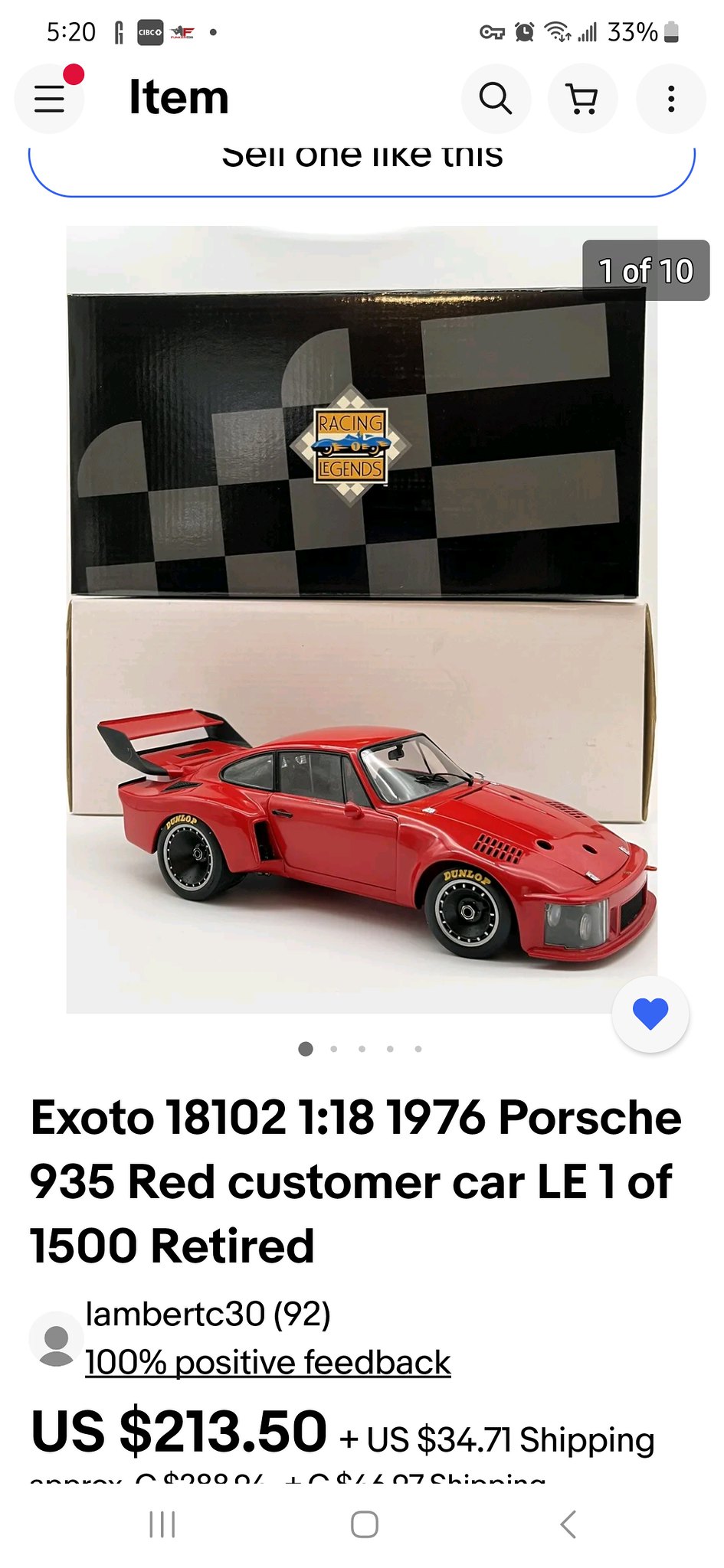In the image, a screenshot from a mobile app showcases a detailed advertisement for a collectible toy car. At the top, the display indicates it's the first of ten images, framed by the current time in the top left corner. Centered prominently is the logo "Racing Legends" over a black and gray checkerboard pattern. Below the logo, the focal point of the image is a vibrant red Porsche 935 sports car, distinguished by its large rear spoiler and two-door design. Accompanying the car, a detailed description appears in black text, reading "EXOTO 18102 1:18 1976 Porsche 935 red custom car. LE, one of 1,500 retired". Additionally, there's a username "Lembertc3092" with a note of 100% positive feedback. The price is clearly marked as "US $213.50" with an additional shipping fee of "$34.71". Notably, a blue heart icon is present by the car image, likely indicating a favorite or liked item on the platform.